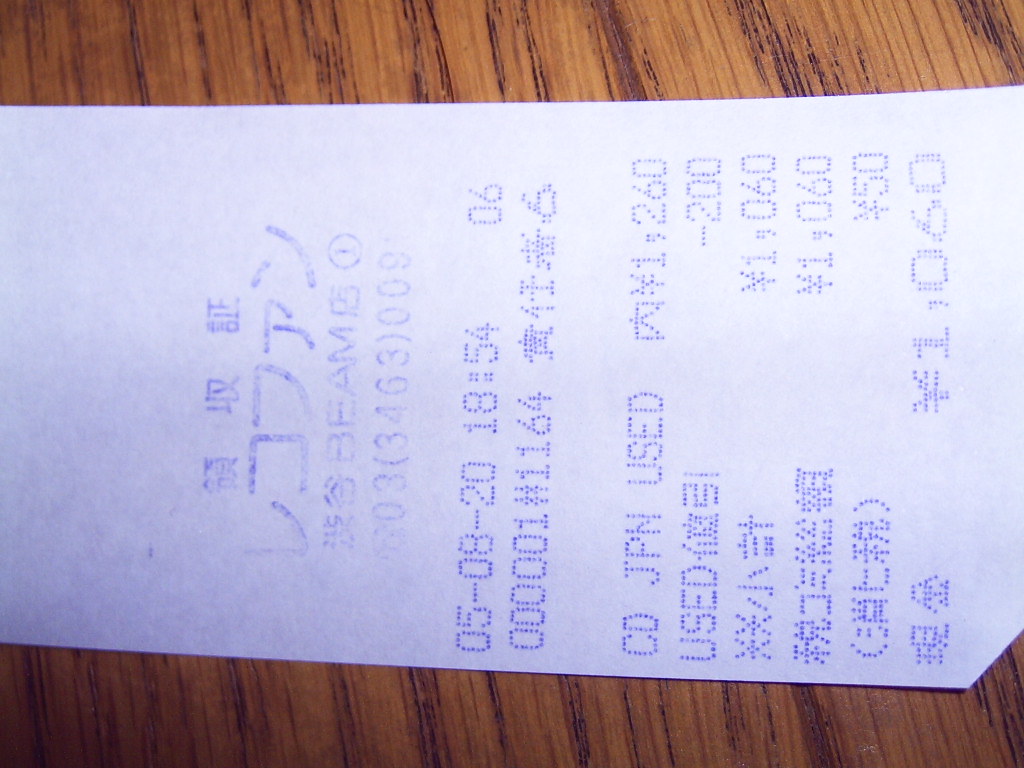The image captures a detailed close-up of a receipt placed on a brown wooden surface. The wooden surface is zoomed in so closely that it's difficult to determine whether it's part of a table, chair, or counter. The receipt itself is oriented horizontally across the picture and features a clean white section transitioning into a blue section on the right end. The text on the receipt appears primarily in what seems to be Japanese characters. Notably, the word "BEAM" is visible on the receipt. Below that, there are numerical entries, including the dates "05-08-20" and the time "18.54," followed by "06." Further down, there is a combination of Asian letters and English, showing "C-D-J-P-N used" and a price of "1,260." A deduction labeled as "used, minus 200" is noted, and the receipt culminates in a total of "1,060" displayed prominently.